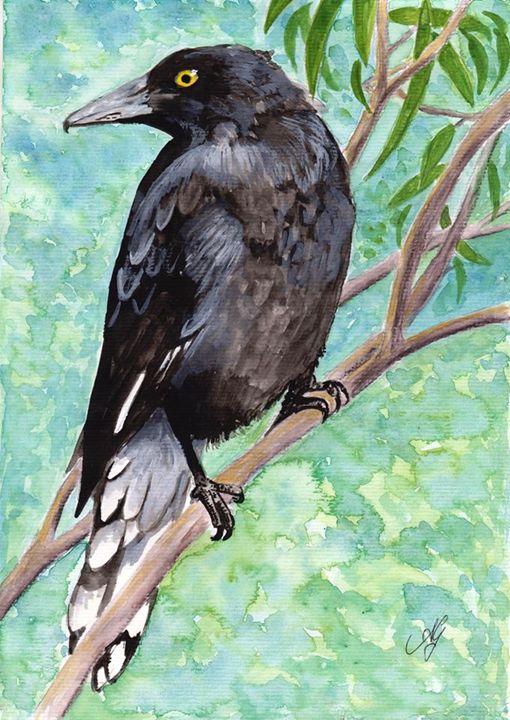This detailed painting portrays a striking black crow perched on a light brown branch that stretches diagonally from the bottom left to the upper right corner of the composition. The background features a splotchy, abstract mix of blues, greens, and whites, reminiscent of a sky. The crow, positioned centrally, displays its chest toward the viewer while its head is turned to look over its left shoulder, showcasing a dark gray-black head, a light black beak, and piercing yellow eyes with black pupils. The bird's plumage is primarily black but blends into gray down its chest, transitioning to white underneath the tail, which points toward the lower left corner and ends in a mix of black and white feathers. The crow's black feet securely grip the branch. Above the main branch and behind the bird, another branch appears, which splits off into three smaller offshoots adorned with dark green leaves. Additional thin branches with green leaves extend into the upper right corner of the painting. A signature by the artist is visible in the bottom right corner, adding a personal touch to the artwork.